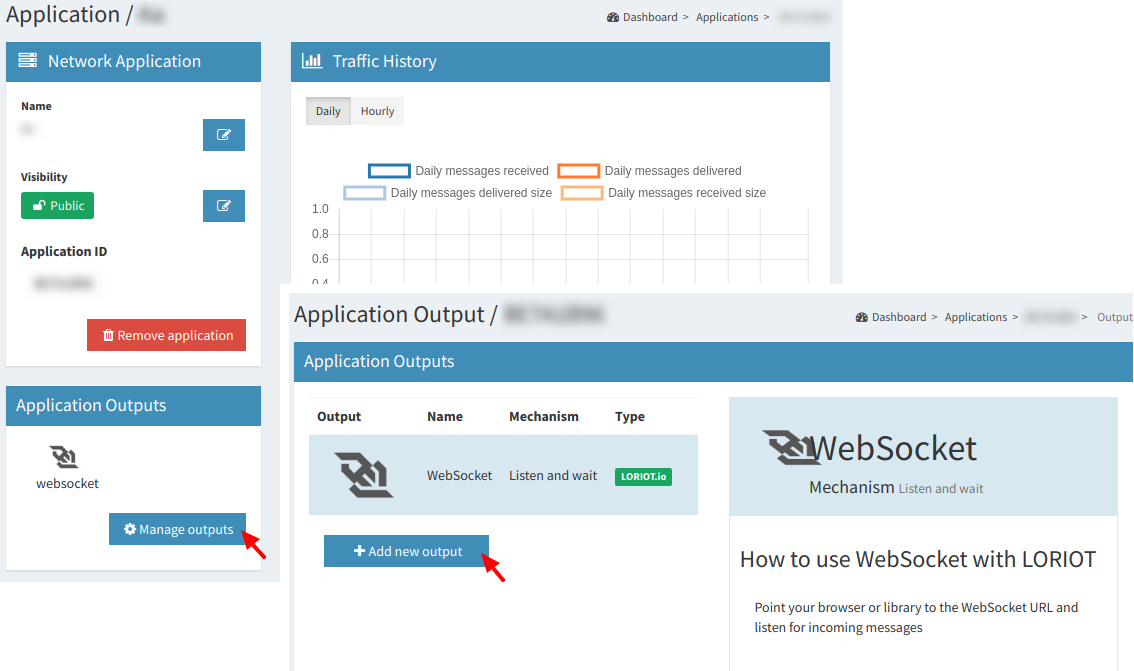The image features a layered view of two webpages, with one prominently displayed in the foreground and the other slightly blurred in the background. The information on both pages has been partially obscured to protect privacy, particularly the phone number and other sensitive details located primarily within a gray strip at the top of the webpage.

The foremost webpage, titled "Application Output," contains blue text underneath that reads "Application Outputs." It provides column headers such as "Output Name," "Mechanism," and "Type." Below these headers, a row displays an emblem followed by the labels "WebSocket," "Listen and Wait," and "Laureate.io." Additionally, there is a highlighted section labeled "Add New Output" in a white font set against a blue background, accentuated by a red arrow pointing to this area.

In the background webpage, which mirrors the layout of the front page, another red arrow directs attention to the "Manage Outputs" section, also distinguished by white text on a blue background.